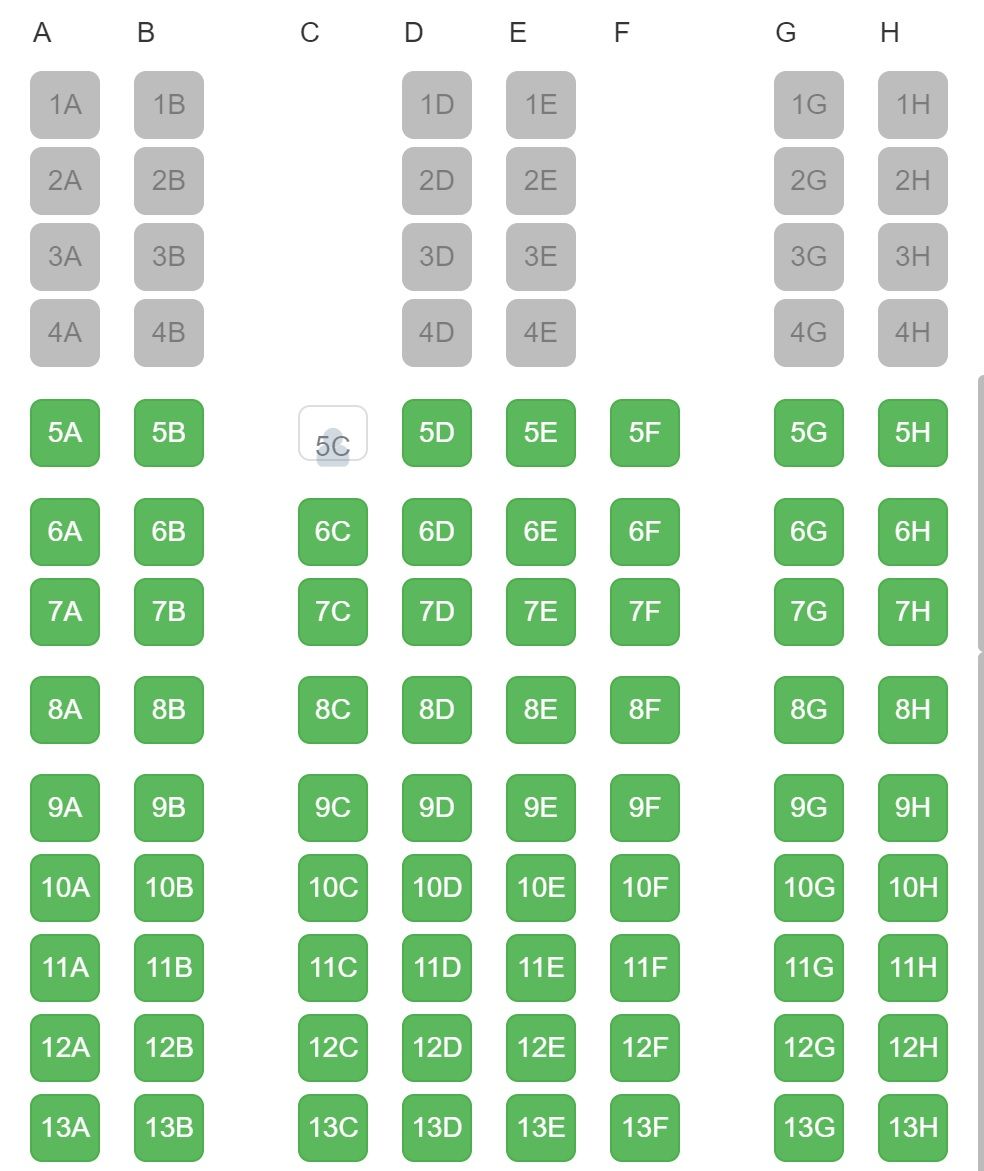This image displays a structured chart against a white background. At the top of the chart, there are black letters spaced out evenly, with "A" and "B" positioned on the left, "C," "D," "E," and "F" in the center, and "G" and "H" on the right. Below these letters are three distinct columns composed of light gray squares with rounded corners. Each column holds four gray squares labeled with a combination of numbers and letters, such as "1A," "1B," "2A," and "2B."

Beneath these gray sections, the format of the chart transitions to green squares, also with rounded corners, filling the remainder of the page. These green squares are marked with white numbers and letters. On the left, the sequence begins with "5A," "5B," and continues similarly. In the center region, there are four columns of green squares following the sequence, including labels like "5C," "5D," "5E," and "5F." On the right side, the chart features two columns with sequences such as "5G," "5H," and so forth.

This organized array creates a visually intriguing pattern, though the purpose or specific context of the chart remains unexplained.